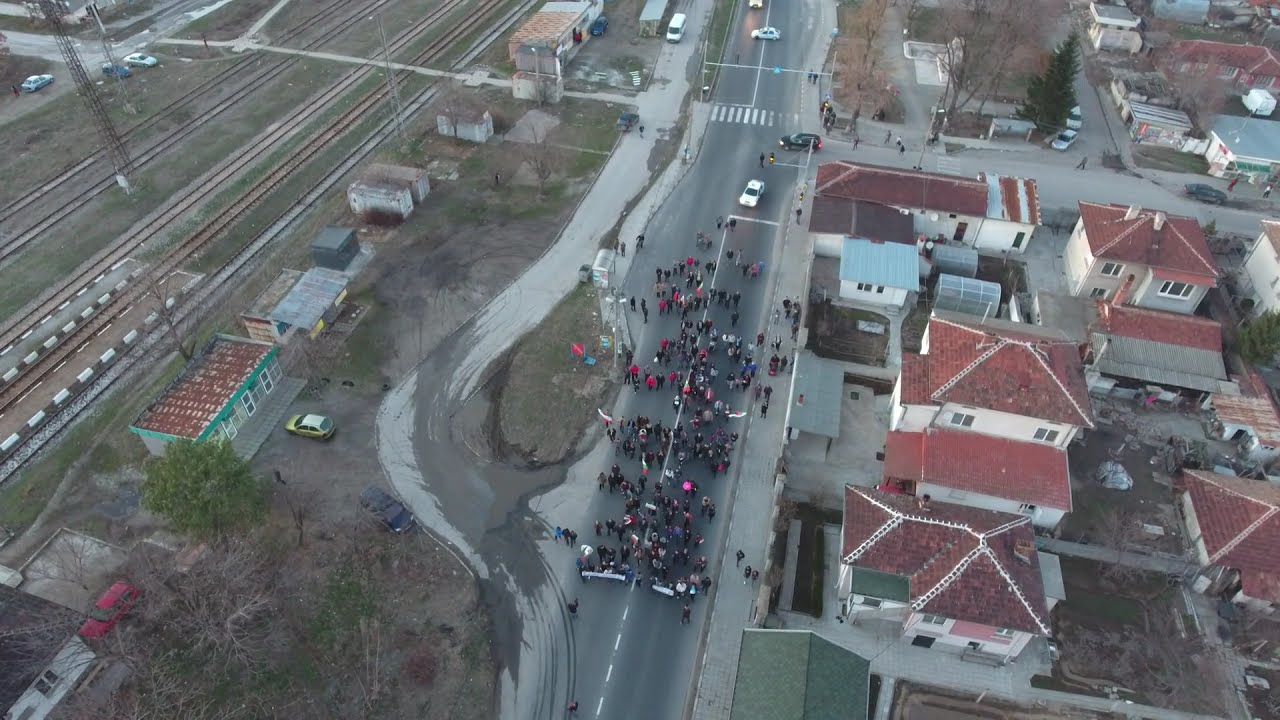This overhead, daylight aerial photograph captures a dynamic scene of a march or demonstration taking place in a small town. The town features predominantly white residential buildings with characteristically red-tiled roofs. The blacktop road, running from the bottom to the top of the image at a slight angle, is marked by a broken white line down the center, designating it as a two-lane road. Approximately 100 people, diverse in size and attire, are marching along this road, holding signs and banners. They are observed proceeding from near the middle of the image towards the top, implying downward movement relative to the photograph.

To the left of the demonstrators, there are five visibly parallel railroad tracks that run from the bottom left to the top left of the image. These tracks are bordered by a secondary road and assorted structures, hinting at a train yard. On the right side of the road are more residential houses, further emphasizing the suburban atmosphere.

At the rear of the procession, the road intersects with another road at a traffic light, where a white car seems to be attempting a turn, followed by a black car. Additional details include an island-shaped section with a red marker or flag situated to the left of the main road, enhancing the map-like perspective created by the drone photography. Overall, the image vividly portrays the bustling activity of a communal demonstration set against the backdrop of a quaint, orderly town.